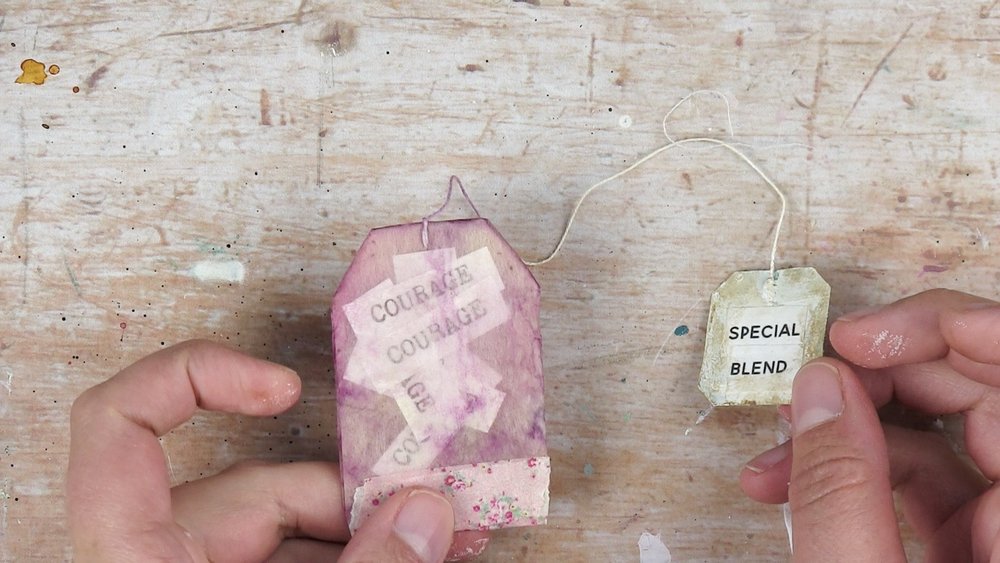In the image, a pair of hands are seen holding two connected pieces of paper resembling teabags against a worn, beige wooden background adorned with dark scratches. The left hand, visible with a forefinger and thumb clasping a larger, six-sided paper slip shaped like an elongated rectangle curved at the top, is filled with several thin strips of paper bearing the word "courage" in black letters on a white background. Attached by a thin white string, the right hand holds a smaller paper slip that says "SPECIAL BLEND" in all-capped black letters. Both hands are positioned at the bottom left and right of the image, displaying clean, straight nails. The teabags are centered slightly towards the bottom of the frame, suggesting the setting might be in someone's home, possibly at a computer desk or similar wooden surface.